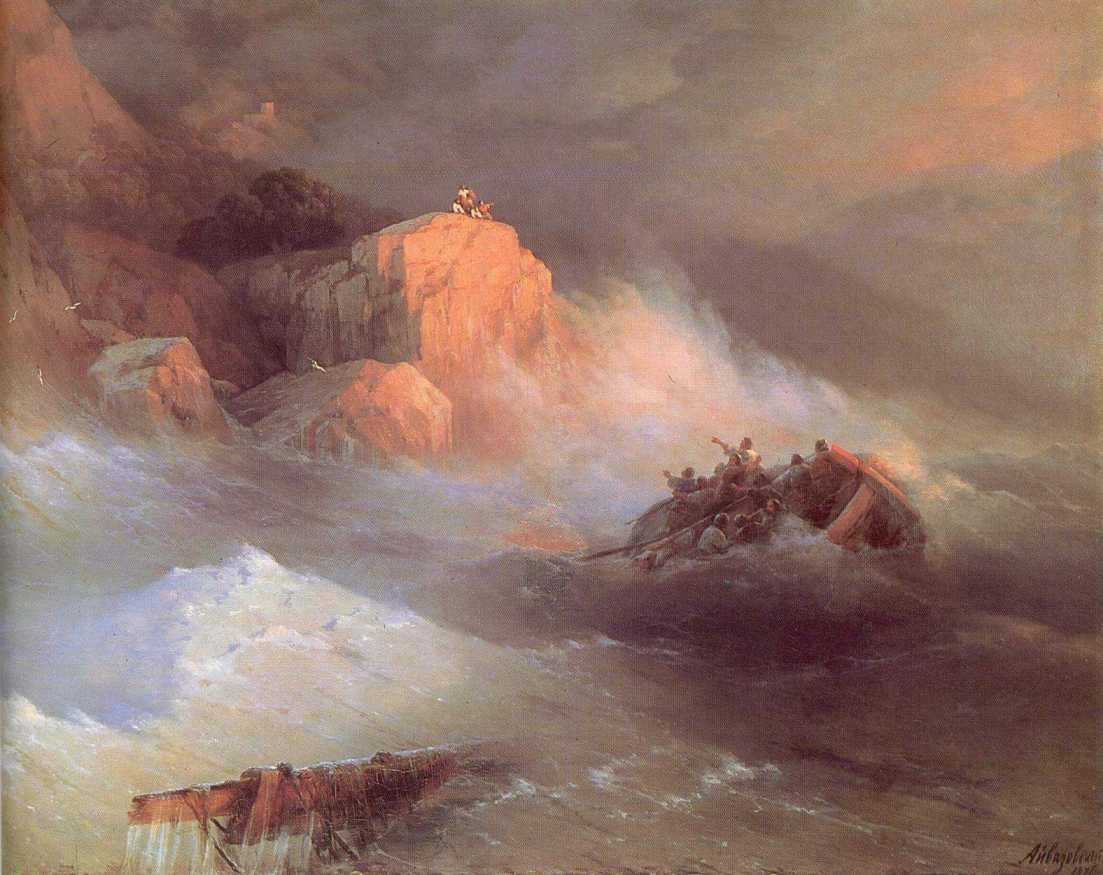The painting, seemingly an oil piece from 1647 signed by A. N. L. A. G. O. B. R. A. N, captures a dramatic maritime scene. Dominated by grim shades of gray, brown, and dark blue with touches of white and reddish-orange, the square composition vividly portrays rough seas against a rocky coastline. To the left, the jagged cliff towers high, sharply descending to the frenzied waves. At its peak, several figures in light clothing peer down toward a perilous scene below. A distressed rowboat, nearly tipping, struggles amidst the tumultuous waters in the middle right section. The occupants gesture frantically toward the figures above, seeking rescue or assistance. Amidst this chaos, remnants of the ship, including a broken mast, float ominously in the churning sea near the lower left. White-capped waves crash viciously against the rocks and vessel, enhancing the sense of urgency and danger in the scene.